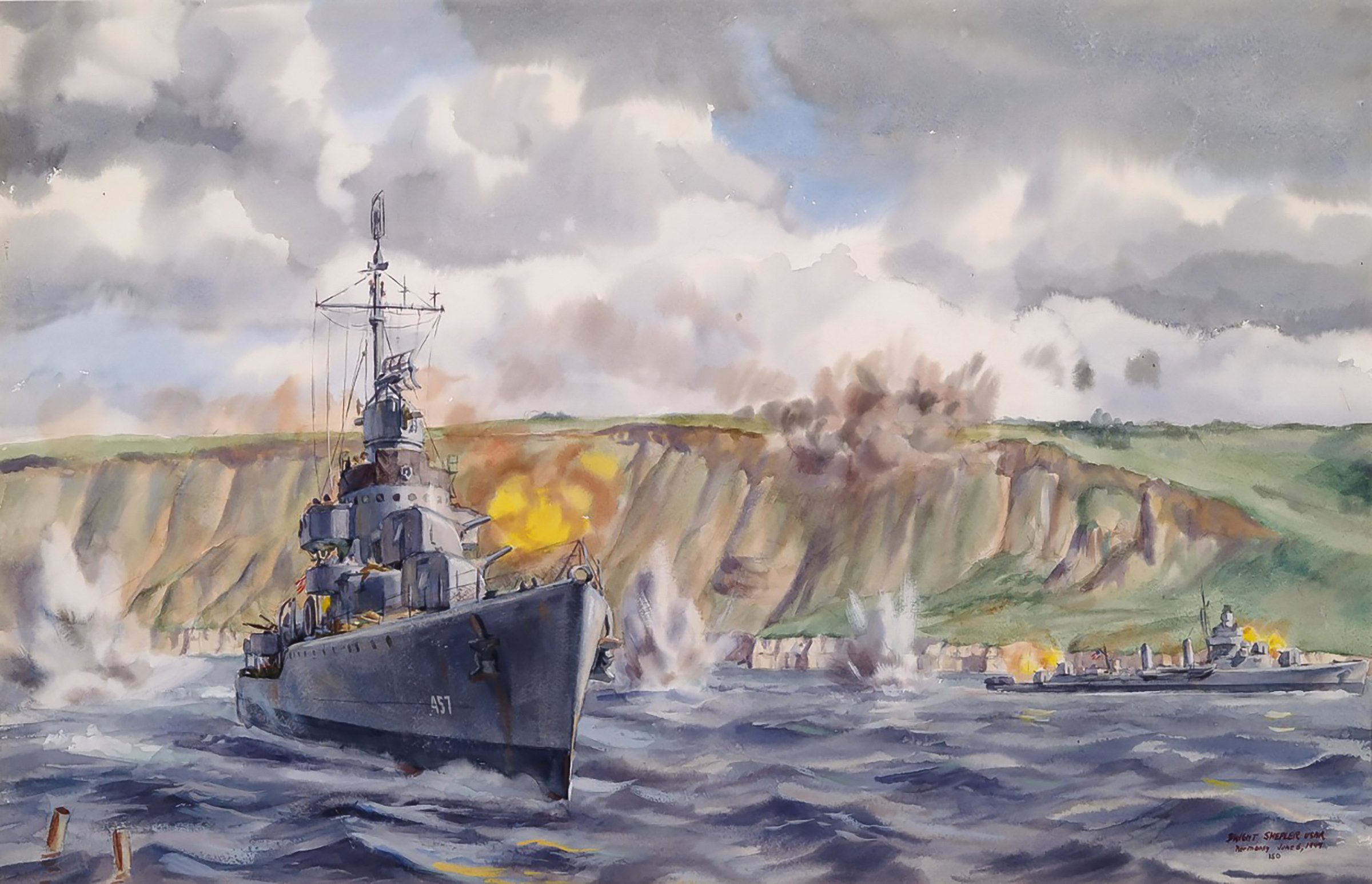The painting vividly portrays a dramatic naval battle scene with two prominent warships engaging on the high seas. In the foreground, a detailed military battleship, possibly made of aluminum with the number 451 painted on its side, dominates the composition. Its tall mast stands out and a puff of yellowish smoke indicates an active cannon firing. The realistic depiction of the cannon fire integrates brilliant hues of orange and red, implying a fierce exchange with the distant ship. The secondary ship, slightly further away, also appears to be discharging its weapons, characterized by similar orange-gold muzzle flashes.

The battle unfolds against a visually striking backdrop, where rugged cliffs and verdant land stretch out in the distance, hinting at a coastline close to an actual country. Unique elements like buildings on the cliffs add further depth and realism to the scene. The ocean below is turbulent, punctuated by splashes where bombs seem to have detonated. The blending of watercolor textures creates a captivating mix of sea, land, and explosive action, highlighting the chaos and intensity of the naval warfare.